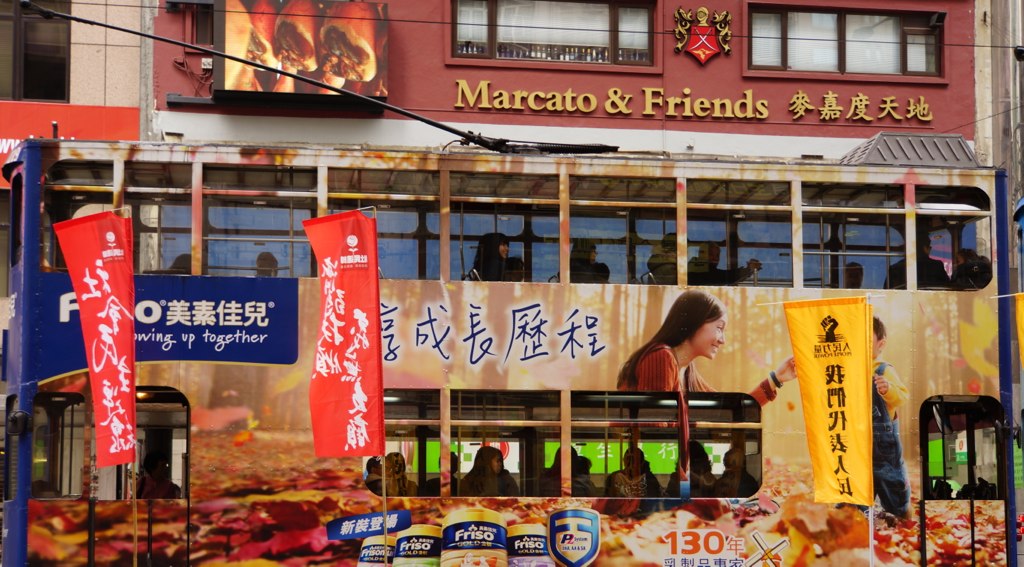The vivid full-color image from Asia captures a bustling scene dominated by a red trolley or bus adorned with vibrant advertisements. At the very top, there's a prominent coat of arms. The building behind it is primarily red, featuring gold printing that reads "Marcato and Friends" alongside Asian text. The trolley is lined with windows through which various passengers can be seen, some looking out. The side of the trolley showcases a large advertisement displaying a woman, trees, and several grocery items, including meats. The front of the trolley is marked with black Asian print, and a black cable car rod is visible. Red and yellow banners with Asian writing hang down, contributing to the scene's lively atmosphere. The area looks somewhat worn, and there's a storefront in the background. To the right of the windows, there's an unclear poster with orange and yellow hues, possibly depicting flames. The surrounding environment suggests a part of town that has seen better days, adding a layer of history and character to the image.